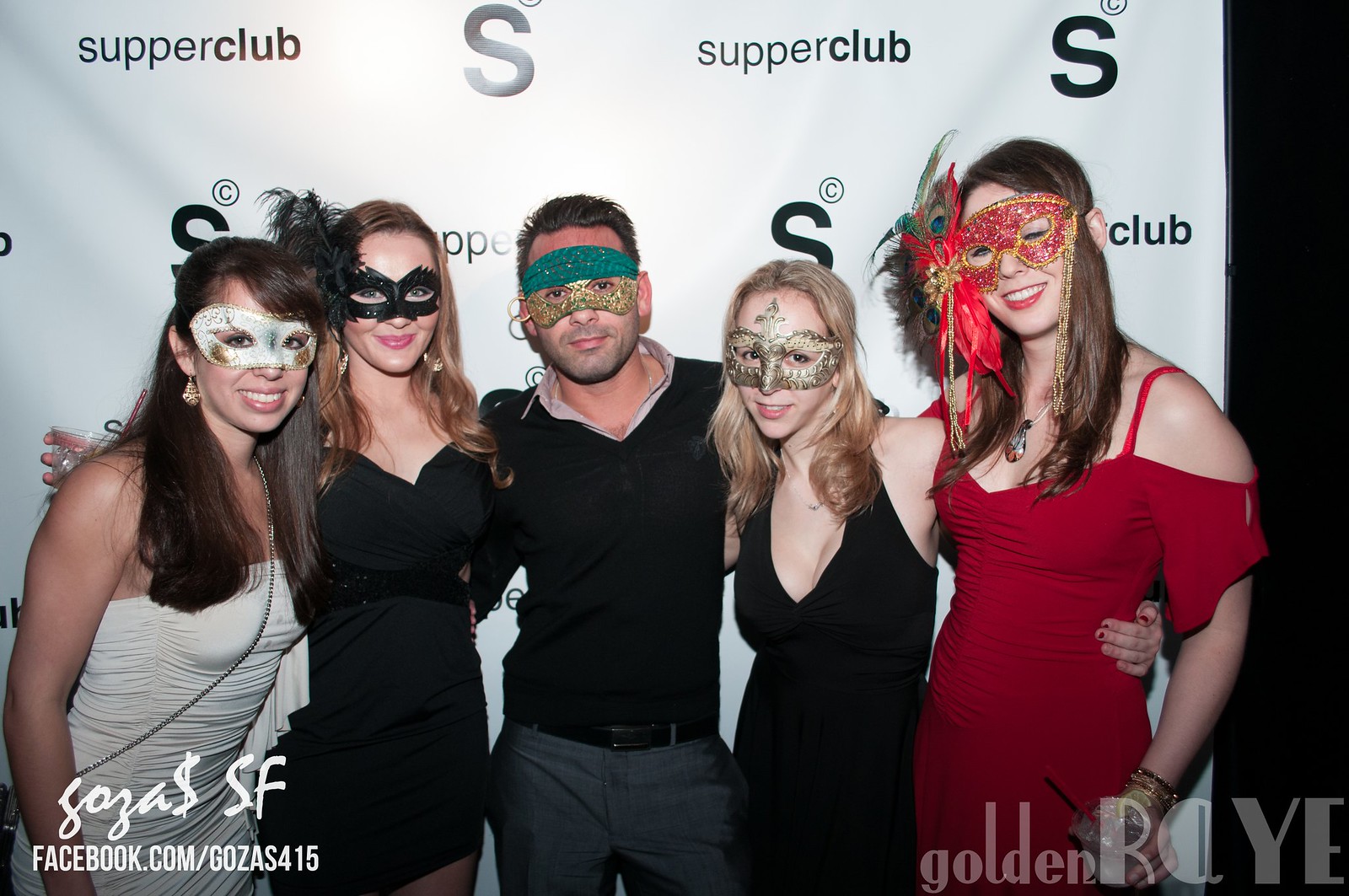Five people, dressed in elegant attire and masquerade masks, are posing in front of a predominantly white background adorned with the repeated text "Supper Club" along with scattered letters "S" and the phrase "Gorja SF" followed by "Facebook.com, Goza S415." From left to right, the first person is a woman in a strapless white dress with a silver mask, long brown hair, and earrings. Next to her is a woman with long, dirty blonde hair in a black dress and a matching black mask. At the center stands a man with short brown hair, dressed in a black sweater and charcoal-colored dress pants, wearing a green and gold mask. To his right is a woman in a black halter dress with shoulder-length blonde hair and a gold mask. The final person is a brunette woman in a red dress, donning a red mask with intricate designs and feathers, winking at the camera.